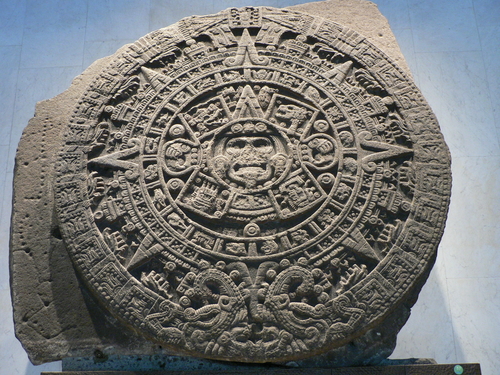The image depicts a detailed, circular stone carving set against a blue sky background. The artifact, which appears broken off from a larger structure, is an intricate representation possibly associated with the Aztec sun stone or calendar. The stone is concrete in color and features a series of concentric circles, each adorned with progressively elaborate designs, including V shapes, circles, squiggly lines, and possible animal heads. The centerpiece of the stone features a prominent, distorted face—reminiscent of a skull—flanked by decorated elements such as extension-like ears and decorations above the head. The outermost edges of the carving are jagged, punctuated with numerous triangular points and arrows that mimic the look of a compass or sun. The base of the artifact includes possible serpent motifs, adding to its complexity. This item might be displayed on a pedestal, likely in a museum setting, given the white tile backdrop. The entire stone is a testament to the detailed and enigmatic artistry linked to ancient Mesoamerican cultures, whether Aztec or Mayan.